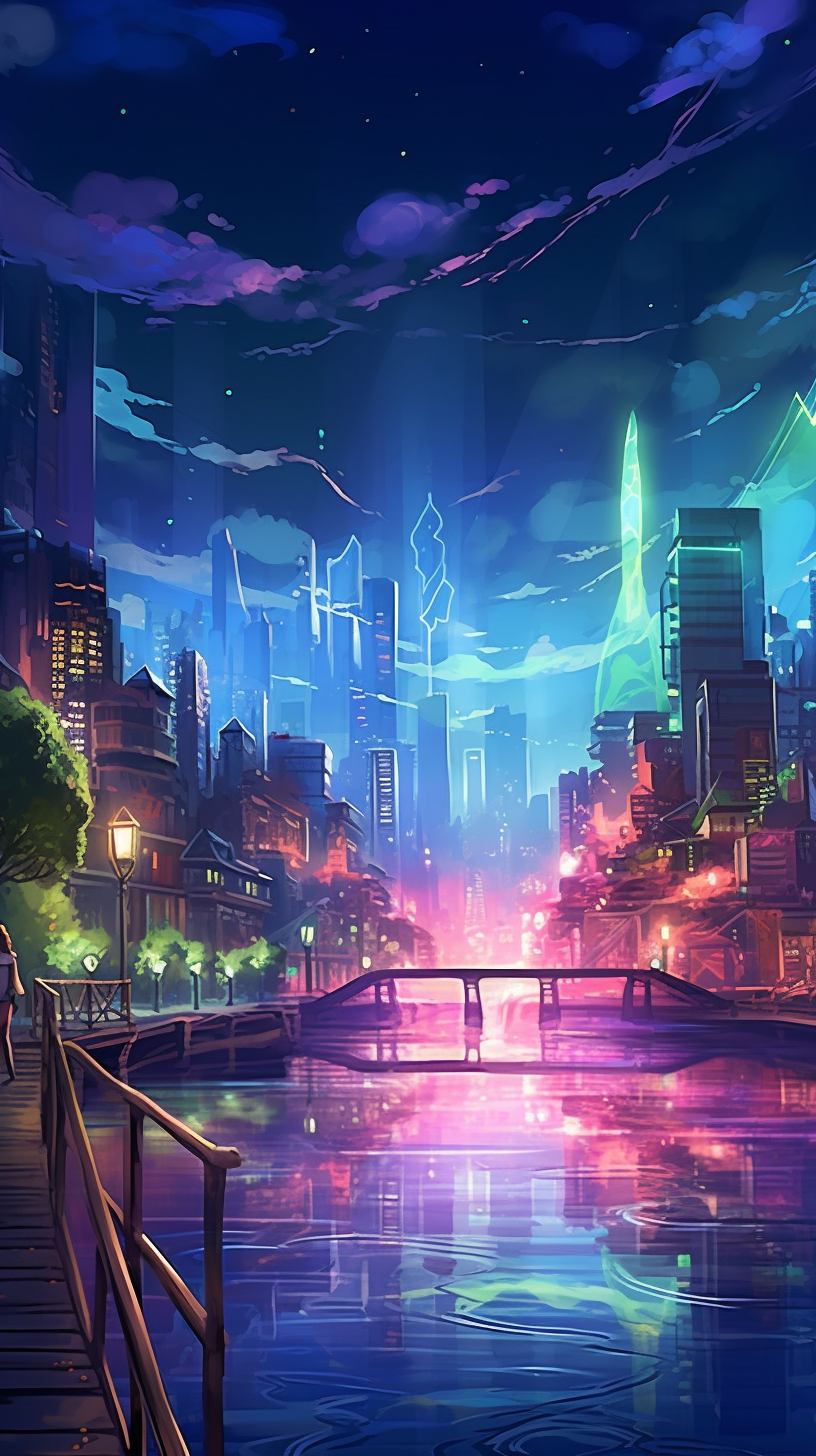This digitally crafted graphic design presents an enchanting nighttime cityscape, brimming with vibrant colors and a fantastical ambiance. Predominantly featuring tones of pink, purple, blue, and green, the artwork displays a meticulous blend of traditional and futuristic elements. At the center of the composition, a footbridge arches gracefully over a waterway, its surface rippling with colorful reflections from the illuminated surroundings. 

On the left, a wooden walkway adorned with glowing lamplights snakes along the water's edge, contrasted by Japanese-style wooden buildings that exude a sense of timeless tradition. In the foreground, green trees add a touch of natural serenity to the scene, while the skyline in the background is dominated by towering skyscrapers bathed in neon pinks and other vivid hues, suggestive of a cyberpunk aesthetic. The dark sky above is beautifully streaked with purple and blue, studded with stars, augmenting the dreamlike quality of the setting. This image, potentially a computer-generated graphic or a screenshot from a video game, masterfully merges elements of urban modernity and artistic fantasy.